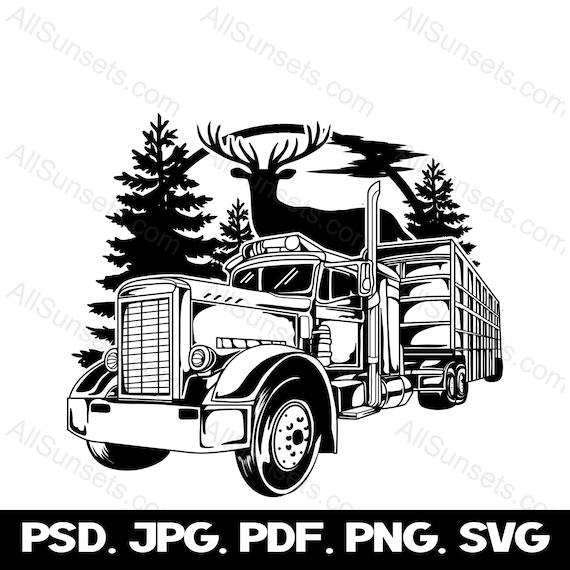This image, watermarked with "AllSunsets.com," depicts a detailed black and white vector illustration available for purchase and commercial use. The central focus is a large 16-wheeler truck hauling a container, set against a backdrop of pine trees and a large celestial body—either the sun or the moon—with small clouds before it. A gigantic deer with impressive antlers stands imposingly behind the truck, gazing upwards. The image also features a thick black bar at the bottom displaying various file format options: PSD, JPG, PDF, PNG, and SVG.